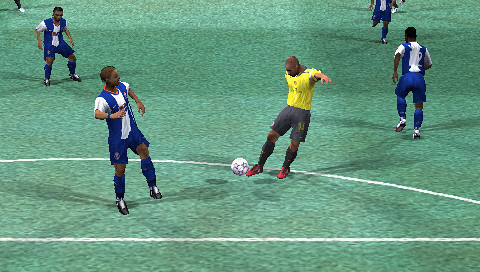This image captures a screenshot of an early, rudimentary soccer video game, apparently a vintage version of FIFA or a similar title. The graphics are noticeably outdated, with clunky and poorly rendered characters on a very flat, green field that lacks texture and depth. Central to the scene is a player in a bright yellow shirt and gray shorts, poised to kick a soccer ball. He stands out with his red cleats amidst a group of four opposing players dressed in blue and white shirts, blue pants, and black cleats. On the periphery, partial figures are visible: in the upper left, the leg of another player can be seen, and in the upper right, about 85% of another player is present. The action is concentrated near white field markings, hinting at a location close to the goal. One blue-clad player near the yellow-shirted character appears to be aiming to intercept the ball, while another in the immediate vicinity seems to be running away. In the background, two more blue-and-white players are converging on the scene, drawn towards the ball and the yellow-shirted player with a focused intent.